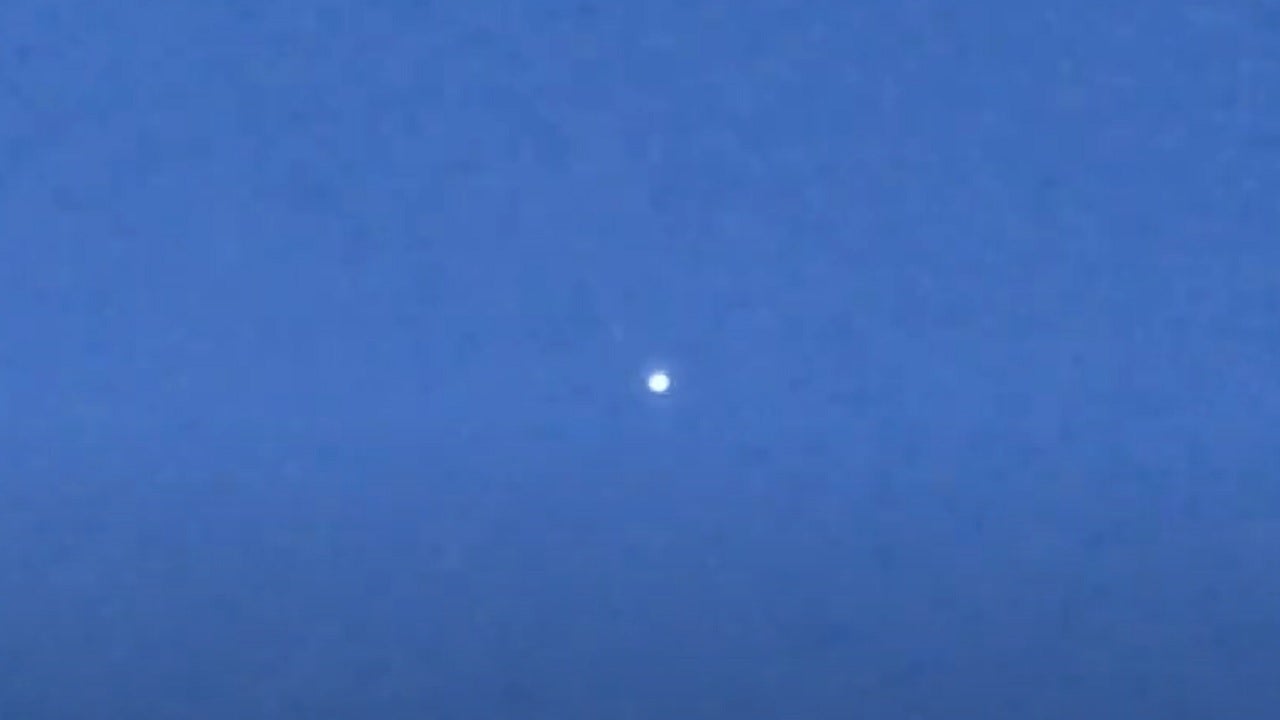In this night-time photograph, taken not long after sunset, the sky has adopted a magnificent gradient of blue that ranges from deep, almost navy hues at the bottom to a richer, vivid blue as you look higher. The image's backdrop captures this transition beautifully, which is characteristic of early evening shots taken with a cell phone. The focal point of the image is a blurry, irregular white dot situated in the center – likely the moon captured from a distance. This slightly out-of-focus celestial body exhibits a faint halo and an uneven shape, emphasizing the challenges of night photography with a mobile device. The interplay of light and the technical qualities of the camera result in a subtle pixelation effect, rendering patches of darker and lighter blues that add a textured, almost surreal aesthetic to the scene.